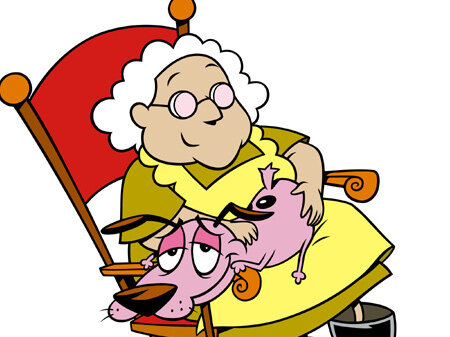The image is a close-up cartoon portrayal of an endearing moment between a grandmother and her dog. The grandmother, an elderly woman with short, bushy, white hair resembling cotton balls, sits contentedly in a red wooden rocking chair, which features two orange circles at the top of its back. She wears large, solid white glasses that obscure her eyes and a soft, pleased expression. Dressed in a lime-green, short-sleeved dress beneath a yellow apron with lighter yellow ruffles, she appears cozy and nurturing. Her legs are adorned with black rain boots, though only their tops are visible. Resting on her lap is Courage, the Cowardly Dog from early 2000s Cartoon Network fame. Courage, depicted as a funky, slightly scruffy purple dog with large, cushiony pink eyelids and a big flat brown nose, lays blissfully on her lap, exuding happiness with a broad smile. His head rests on the wooden arm of the rocking chair. The background of the image is stark white, drawing full attention to this tender scene.